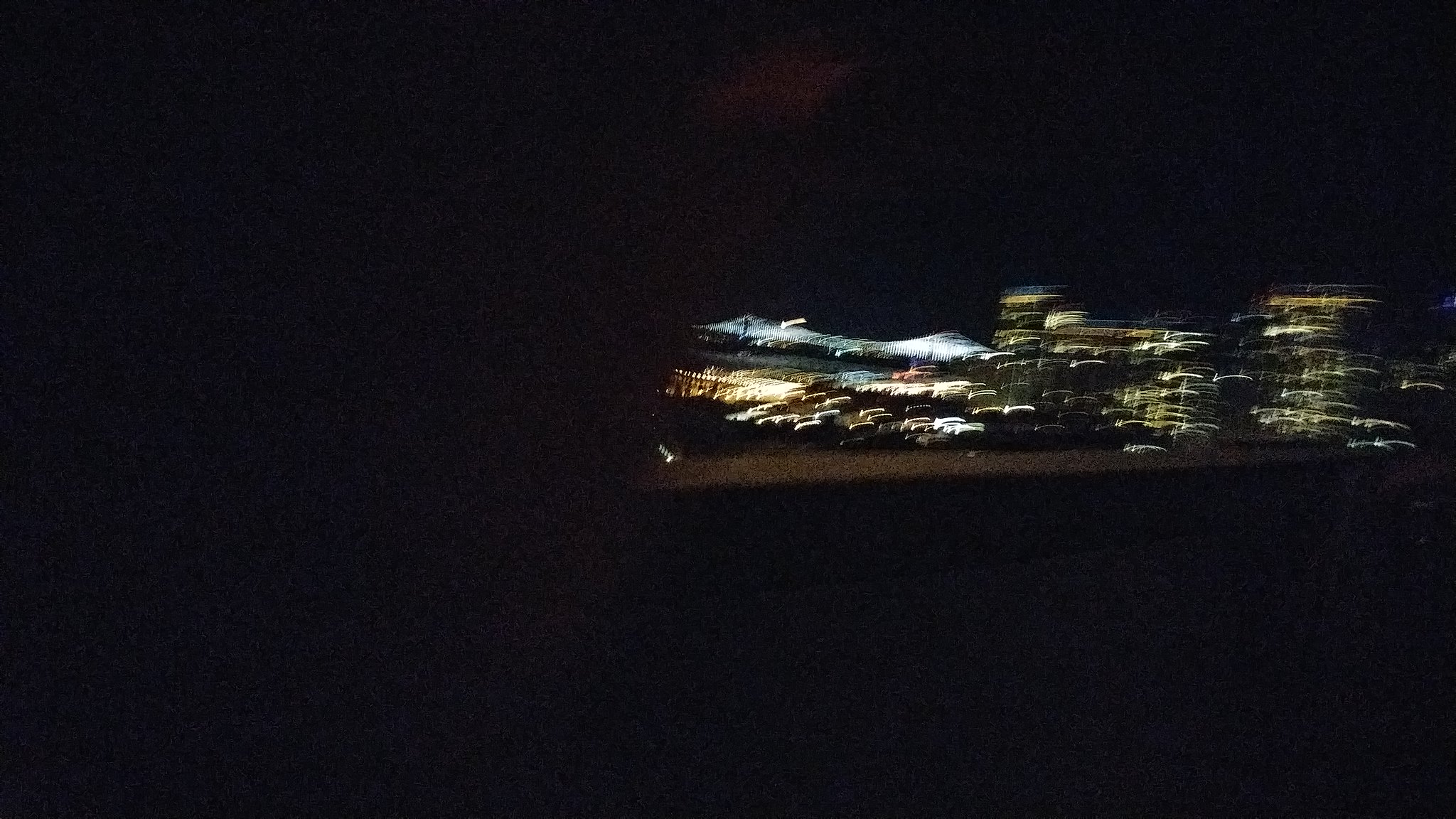A mesmerizing, double-exposed nighttime photograph captures a bustling downtown cityscape in all its hazy glory. The image, taken horizontally, prominently features a cluster of five tall buildings outlined against the horizon. To the left, a suspension bridge bathed in a crystal-blue light adds a touch of architectural elegance. The cityscape, seen from a vantage point that appears to be another bridge in the foreground, reveals a mosaic of lower buildings beneath the towering skyscrapers. The double exposure effect causes the city lights to streak across the image, creating a dynamic and slightly surreal effect. The foreground is enveloped in deep shadows, with a mysterious, semi-opaque object—possibly a finger or an obstacle—partially obscuring the lens. The night sky above remains cloaked in darkness, enhancing the enigmatic and moody atmosphere of the scene.